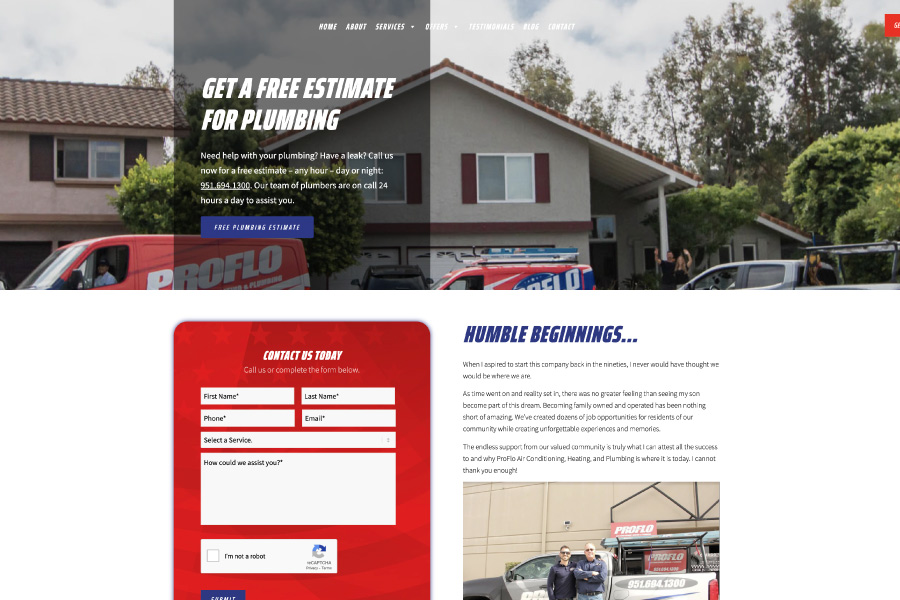On the website, a vivid image captures a house with the company's fleet—a pair of red and blue branded ProFlow trucks—parked outside. The scene is set against a backdrop of lush trees and a slightly overcast sky, hinting at a typical suburban neighborhood with grayish houses. The page prominently promotes a call to action: "Get a free estimate for plumbing" with a prompt for immediate assistance, emphasizing 24/7 availability. The phone number, 951-694-1300, is given for urgent calls.

At the top of the site, navigation tabs—Home, About, Services, Offers, Testimonials, Blog, and Contact—can be seen, albeit with some difficulty due to their white font against the background. Below this section, a bold red banner invites users to "Contact Us Today," providing fields for name, phone number, email, service type, and a text box for detailing issues.

On the right side of the page, a section titled "Humble Beginnings" recounts the company's origin story, featuring an image of two men, presumably the founders, standing proudly next to a car. Behind them, the ProFlow brand is displayed on a red sign. This historical note indicates the company started in the 1990s, grounding its present-day expertise in decades of experience. A blue button labeled "Free Plumbing Estimate" offers a convenient way to request service amidst the detailed, user-friendly layout.